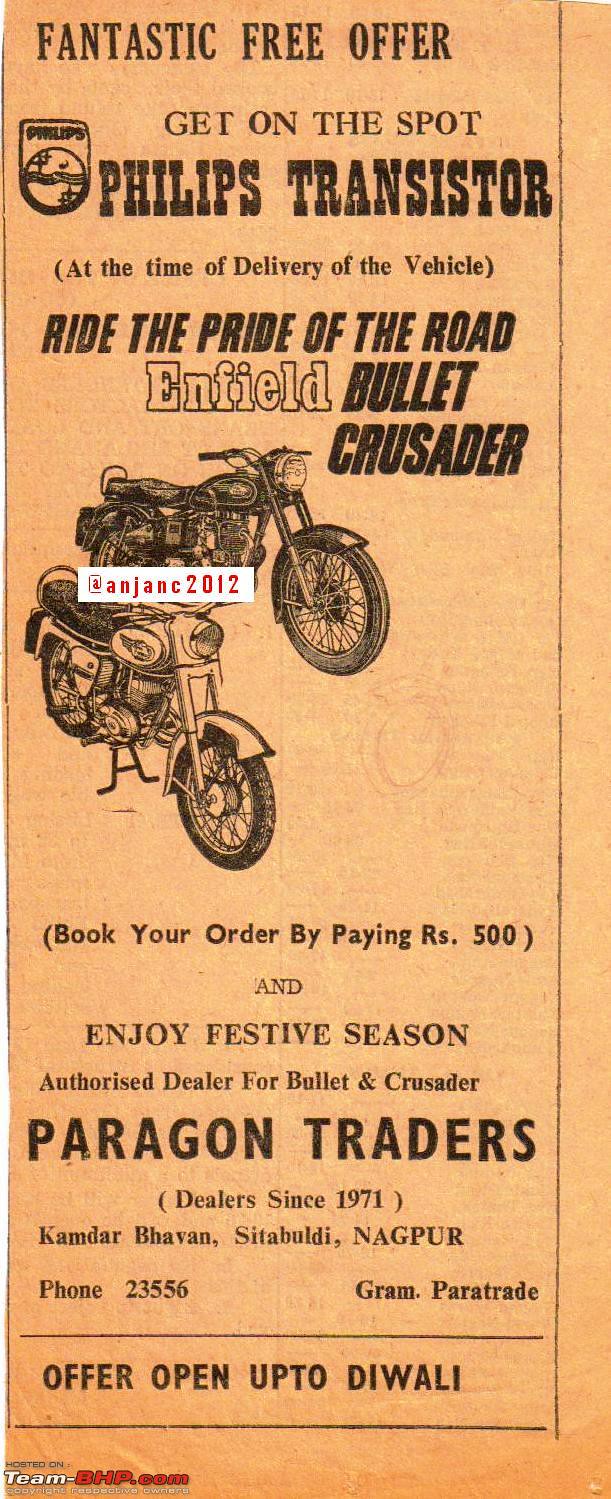This image is a scan of a faded, yellowed newspaper clipping displaying an advertisement for motorcycles, specifically the Enfield Bullet Crusader models. At the very top, in bold black letters against the aged paper, it announces a "Fantastic Free Offer." The ad promotes receiving a Philips transistor on the spot at the time of vehicle delivery, highlighted by the Philips logo to the left. The motorcycles are depicted prominently in the middle, with one appearing slightly larger, possibly due to its position above the other. Text beneath the motorcycles encourages customers to "Ride the pride of the road" with the Enfield Bullet Crusader.

Further down, instructions are provided to "Book your order by paying RS.500 and enjoy the festive season," clearly indicating a celebratory marketing angle, likely aimed at the Diwali season, an important Indian festival. The advertisement mentions Paragon Traders as the authorized dealer, situated in Tamdar Bhavan, Sittibaldi, Nagpur, and features their phone number, 23556. "Since 1971" emphasizes the longevity and reliability of the dealer. The offer is noted to be open up to Diwali. An additional detail includes the term "Graham Paratrad," but its specific relevance is unclear. The lower left corner also contains a web address, "teamphp.com," likely associated with the ad's provenance or related marketing.